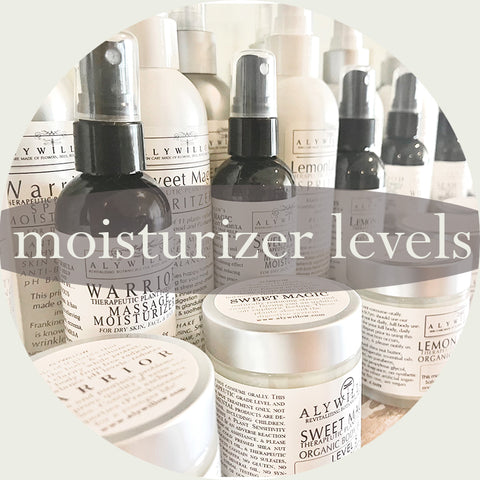The image is an advertisement for body care products with a light gray square frame around it. At the center, a translucent gray oval banner prominently displays the text "Moisturizer Levels" in white font. Inside the circle bordered by the frame, various beauty products are showcased. In the foreground, there are jars with silver caps and white labels featuring dark gray print detailing the product information. Behind the jars, rows of pump spray bottles are arranged: one row features white and silver bottles, while another row includes black spray bottles. The labels on the products have a minimalist design with a lot of text and no images, emphasizing words like Ally, Sweet, Organic, Warrior, Massage, Therapeutic, Moisturizer, and Lemon. The products appear to be organic massage moisturizers available in different scents.